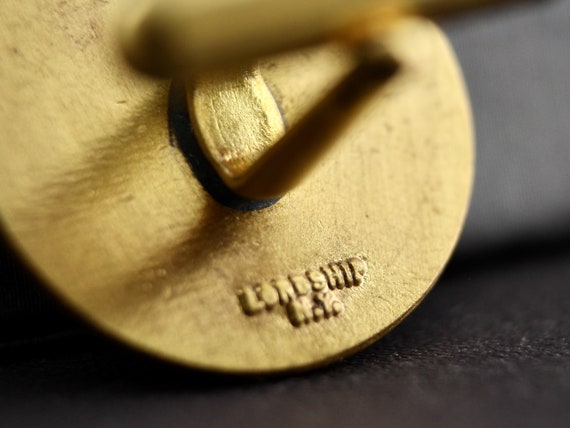This is an intricate close-up of a golden, circular flat disc crafted from a shiny gold-colored metal. The surface of the metal is slightly textured, lending it a rustic, aged appearance that enhances its vintage charm. Embossed upon the disc is the word "LORDSHIP," followed by the letters "N.Y." with periods, indicating New York or possibly a person's initials. A small metallic pin or shaft is partially visible through the center of the disc, suggesting that it might be part of a larger mechanical assembly or a decorative piece. The skillful photography accentuates the meticulous craftsmanship and detail of the embossed text and textured surface, all set against a contrasting grayish-black background.